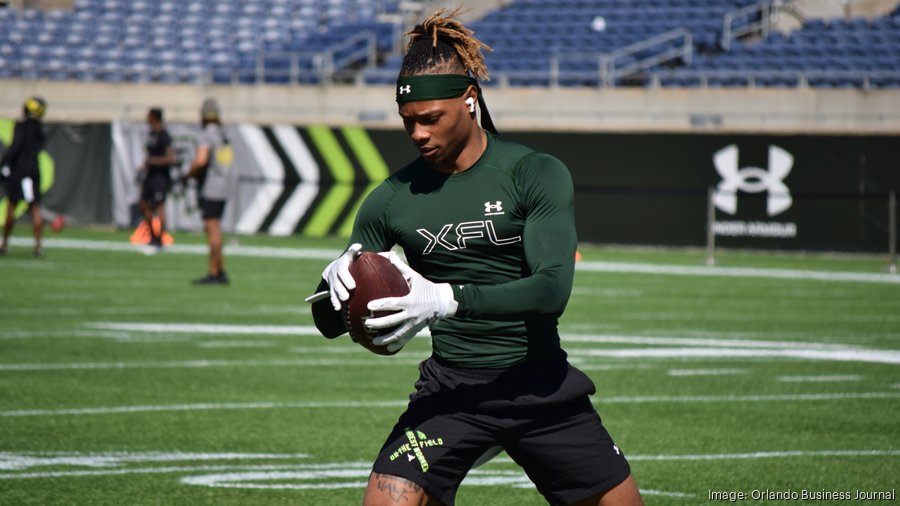The image captures an African-American athlete, likely during a training session on a football pitch. He is the central focus, standing with legs slightly apart, appearing poised to throw a football. His hair is styled into dreadlocks, tied back with an Under Armour headband that matches the dark moss-green, long-sleeved, skin-tight top he is wearing. The top prominently features the XFL logo, suggesting his association with the league. His attire also includes black shorts, which have an XFL logo and an Under Armour brand emblem. He wears pristine white gloves, holding a brown-tan football while looking intently down at it, indicative of deep concentration. 

In the background, the stadium's seating is faintly visible along with advertising for Under Armour. Three other players, likely teammates, are positioned on the pitch behind him. The image is credited to the Orlando Business Journal, adding a touch of authenticity and context to the scene.